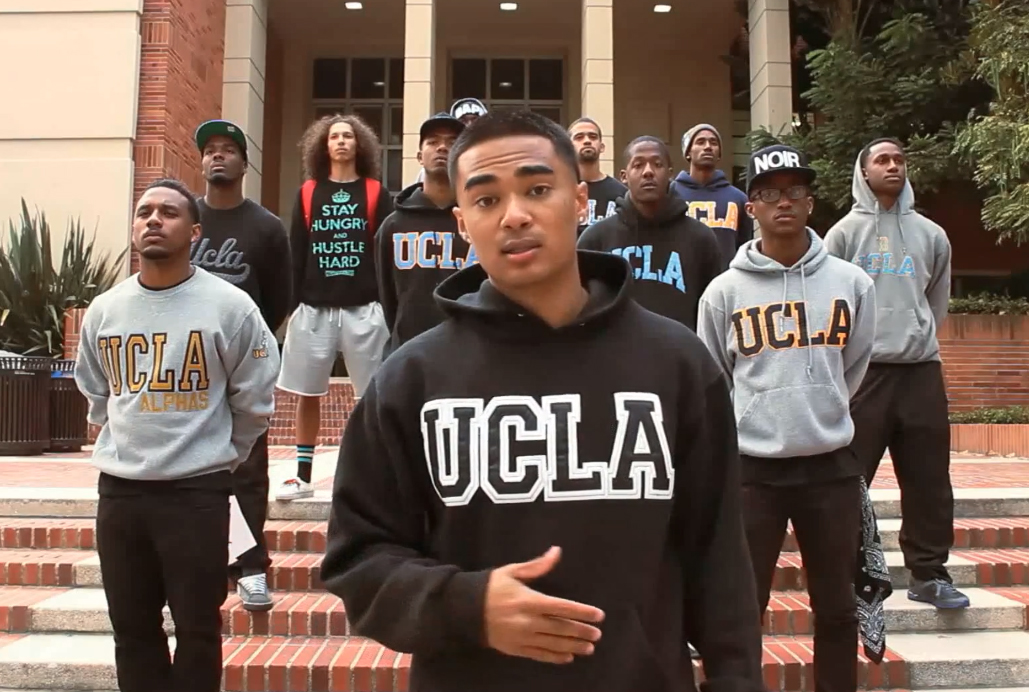The photograph features a group of young African-American men standing on a set of concrete and red brick steps outside a building with concrete and brick accents, likely part of UCLA. The students are arranged in five staggered rows. All but one are wearing UCLA hoodies in various colors, including gray with yellow lettering and black with blue lettering. One man in the back sports a sweatshirt that reads "Stay Hungry and Hustle Hard." The men appear to be in their early twenties.

The man in the foreground, who is positioned closest to the camera, stands out prominently. He has a light skin tone, short-cropped black hair, and brown eyes, suggesting possible Asian descent. His eyebrows are raised, and his mouth is slightly open as though he is speaking, with his right hand gesturing in front of him. His direct gaze at the camera adds a sense of immediacy and engagement, implying he might have just finished addressing an audience. Given the context of the scene, the image evokes the atmosphere of a demonstration or protest, though no placards or visible markers indicate the specific cause.